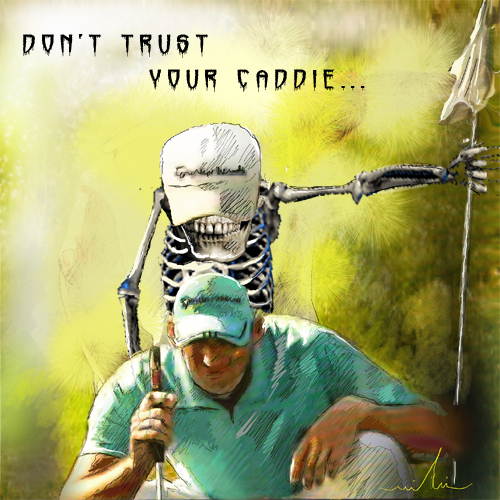The image is a stylized, cartoonish graphic that depicts a golfer in a crouched position, carefully lining up a putt. The golfer is dressed in a light teal green short-sleeved shirt and cap, paired with white pants. He holds a putter in one hand and balances the other on his knee. Directly behind him stands his caddy, who is eerily depicted as a skeleton. The skeleton caddy, with visible teeth, is dressed in a white hat with some writing on it and holds a golf flag. The background features a splotchy yellowish-green texture, enhancing the overall unsettling atmosphere. Above the caddy, in black, dripping, creepy font, the words "Don't Trust Your Caddy..." are prominently displayed. The graphic also includes the artist's signature in the lower right corner.